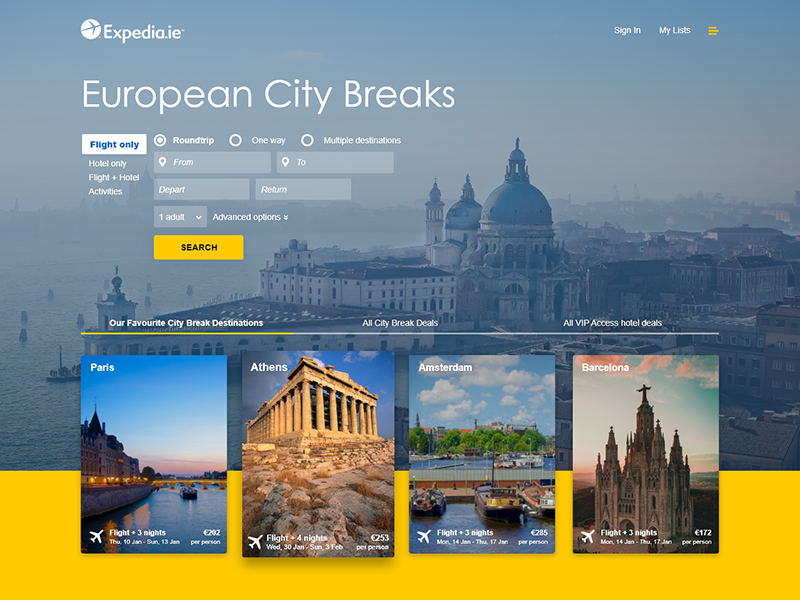This screenshot captures an Expedia.ie webpage, featuring a picturesque aerial view of a European or Turkish city as its background. At the center of the image, there is a prominent domed church surrounded by numerous buildings, all situated along an ocean or bay. Overlaid in white font across the backdrop are the words "Expedia.ie European city breaks." A white rectangular banner below this text features the options: "Flight only" in blue font, "Hotels only," "Flight and hotel," and "Activities" in white font. To the right of "Flight only" are three clickable circles labeled "Round trip," "One way," and "Multiple destinations," with "Round trip" currently selected. Below these options are gray fields for entering departure and destination cities, departure and return dates, and the number of adults traveling. Further down, a yellow rectangle with "Search" written in black prompts users to initiate their booking search. At the very bottom, four smaller photos of cities—Paris, Athens, Amsterdam, and Barcelona—are displayed along with their respective flight prices.